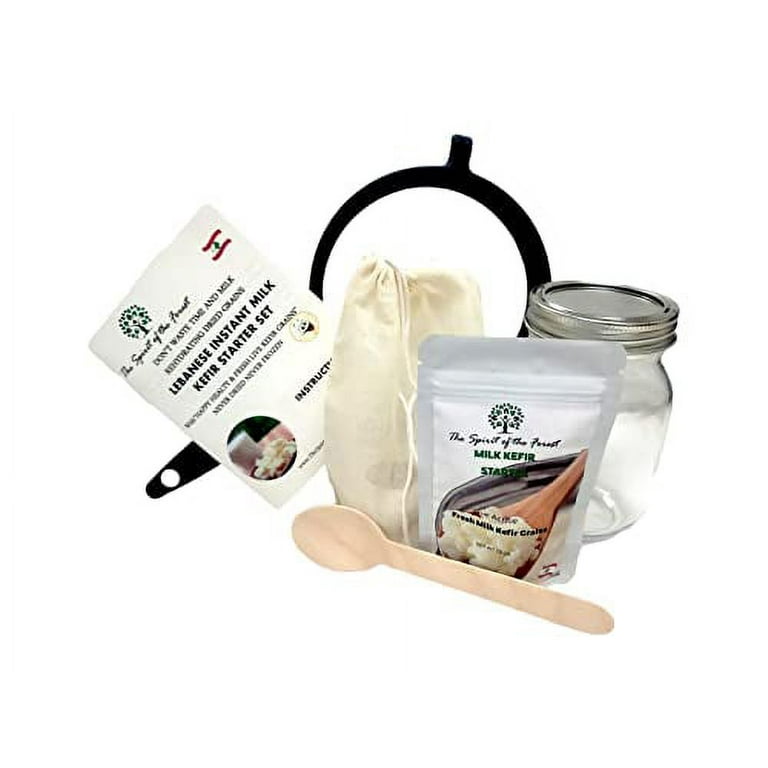The image is a detailed, color photograph of a collection of supplies for making milk kefir, set against a white background. The scene is brightly lit and sharply focused. Prominently on the left, there is a white packet featuring a small green tree in the top left corner and the Lebanon flag, characterized by two red stripes with a green cedar tree in the middle, on the right. This packet is labeled in black text, "Don't waste time in milk, rehydrating dead grains. Lebanese instant milk kefir starter kit." Positioned centrally in the image is a vertical cream-colored bag with a drawstring at the top. In front of it lies a white packet labeled "The spirit of the forest milk kefir starter" with a photo of a wooden spoon filled with a white substance. To the right of this, there is a clear glass mason jar with a silver screw-on lid. A wooden spoon with a light wood color is displayed at the bottom, angled with the handle pointing toward the lower right. Above the wooden spoon, partially overlapping the top of the cream-colored bag, is a black sifter with a handle pointing to the lower left. The overall composition of the items presents a cohesive and organized setup ideal for a product photography style aimed at showcasing kefir making kits in a clear and professional manner.